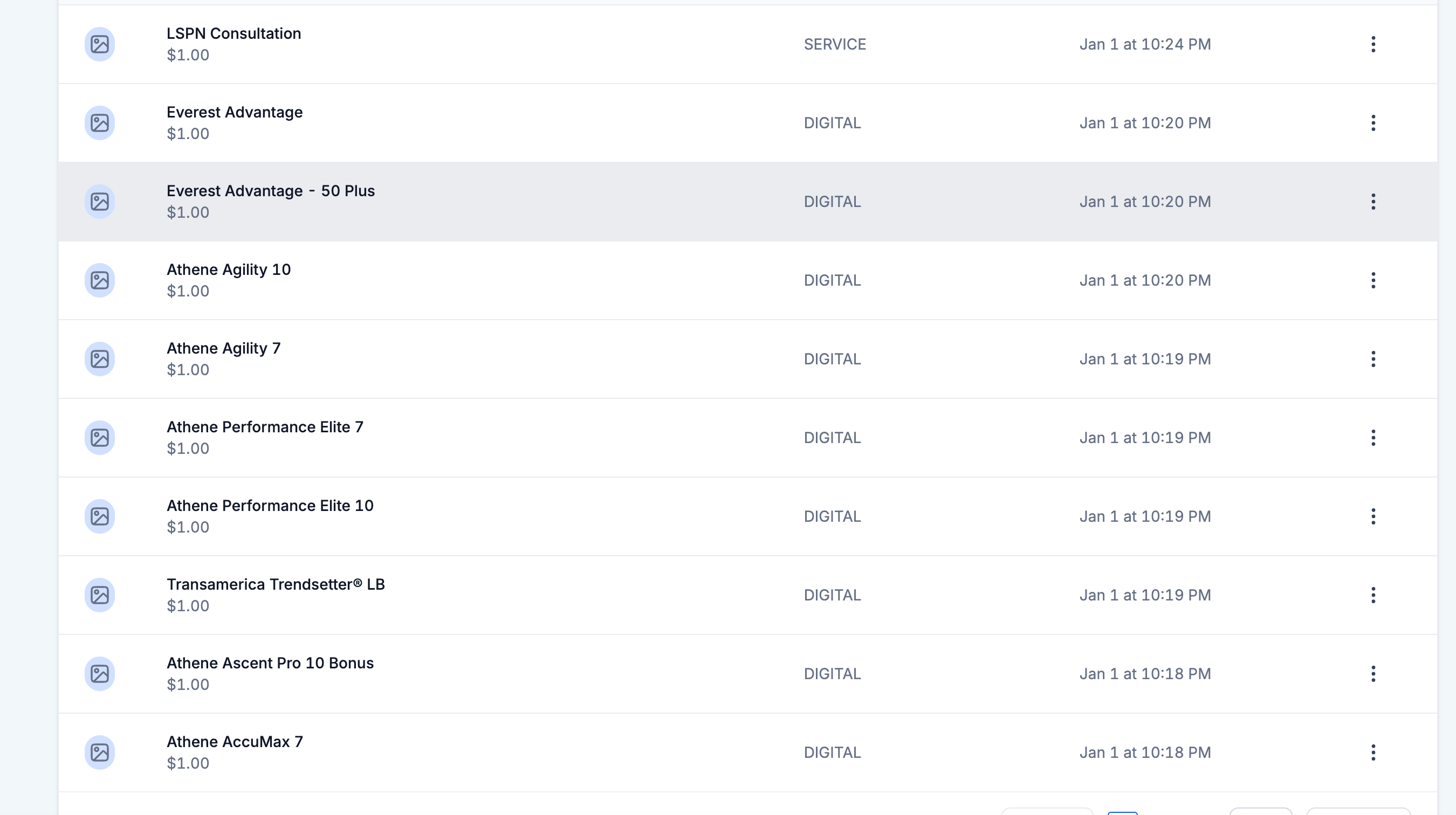This is a detailed screenshot depicting a vertical list of financial or service entries, each contained within individual white rectangles, totaling ten entries. The entries are clearly organized with key details such as service names, costs, types, and timestamps. 

1. **LSPN Consultation**
   - Cost: $1.00 
   - Type: Service
   - Date and Time: January 1st at 10:24 p.m.

2. **Everest Advantage**
   - Cost: $1.00 
   - Type: Digital
   - Date and Time: January 1st at 10:20 p.m.

3. **Everest Advantage - 50 Plus**
   - Cost: $1.00 
   - Type: Digital
   - Date and Time: January 1st at 10:20 p.m.

4. **Athene Agility 10**
   - Cost: $1.00 
   - Type: Digital
   - Date and Time: January 1st at 10:20 p.m.

5. **Athene Agility 7**
   - Cost: $1.00 
   - Type: Digital
   - Date and Time: January 1st at 10:19 p.m.

6. **Athene Performance Elite 7**
   - Cost: $1.00 
   - Type: Digital
   - Date and Time: January 1st at 10:19 p.m.

7. **Athene Performance Elite 10**
   - Cost: $1.00 
   - Type: Digital
   - Date and Time: January 1st at 10:19 p.m.

8. **Transamerica Trend Center LB**
   - Cost: $1.00